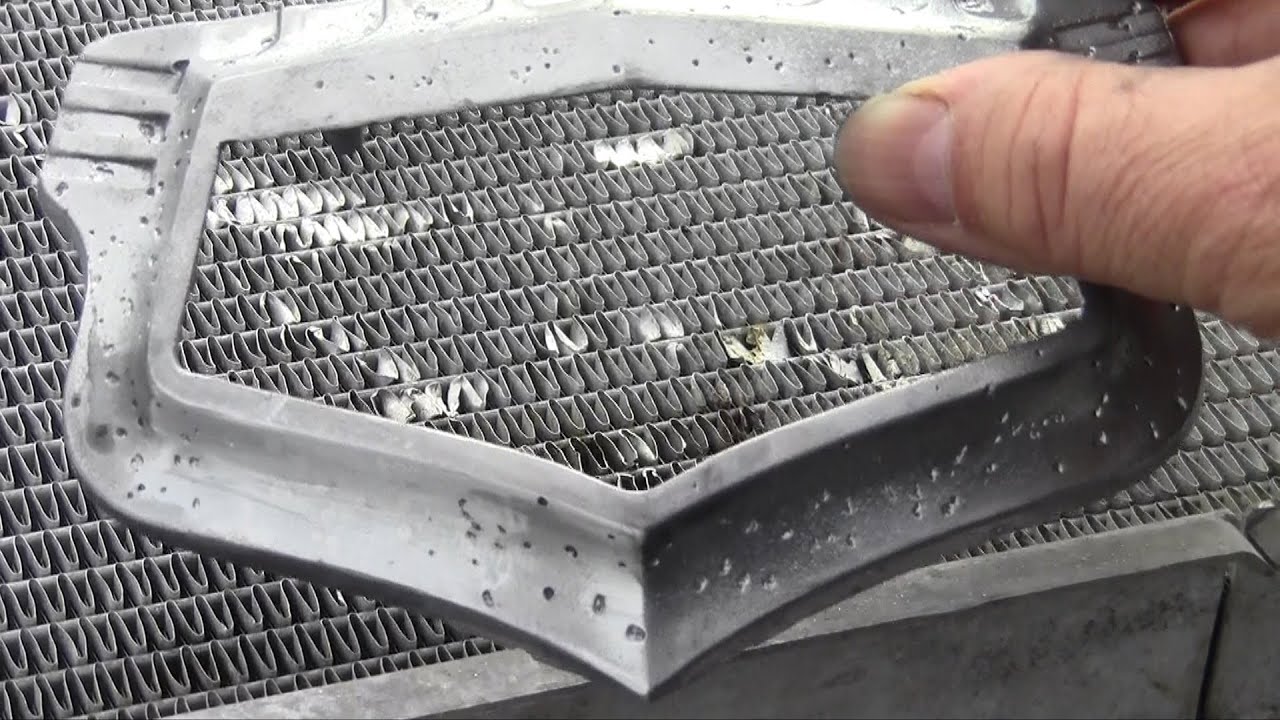In the image, we see the hands of a white male with long, somewhat dirty nails holding a metallic device that resembles a curved shield or emblem. This device, referred to as a holoshield by one description, is being held above a metallic grate. The shield has an empty, hollowed-out space in the middle, and appears to be dented, bruised, and damaged, with numerous tiny holes and brighter spots indicating wear. Its surface also features patterns mimicking wave lines and has three engraved stripes at the top right corners. The grate below the shield has rows of small holes arranged horizontally and shows signs of damage, with some areas pressed down and others appearing partially melted. The entire setup could be reminiscent of a car emblem being placed against a detailed and worn metallic background.